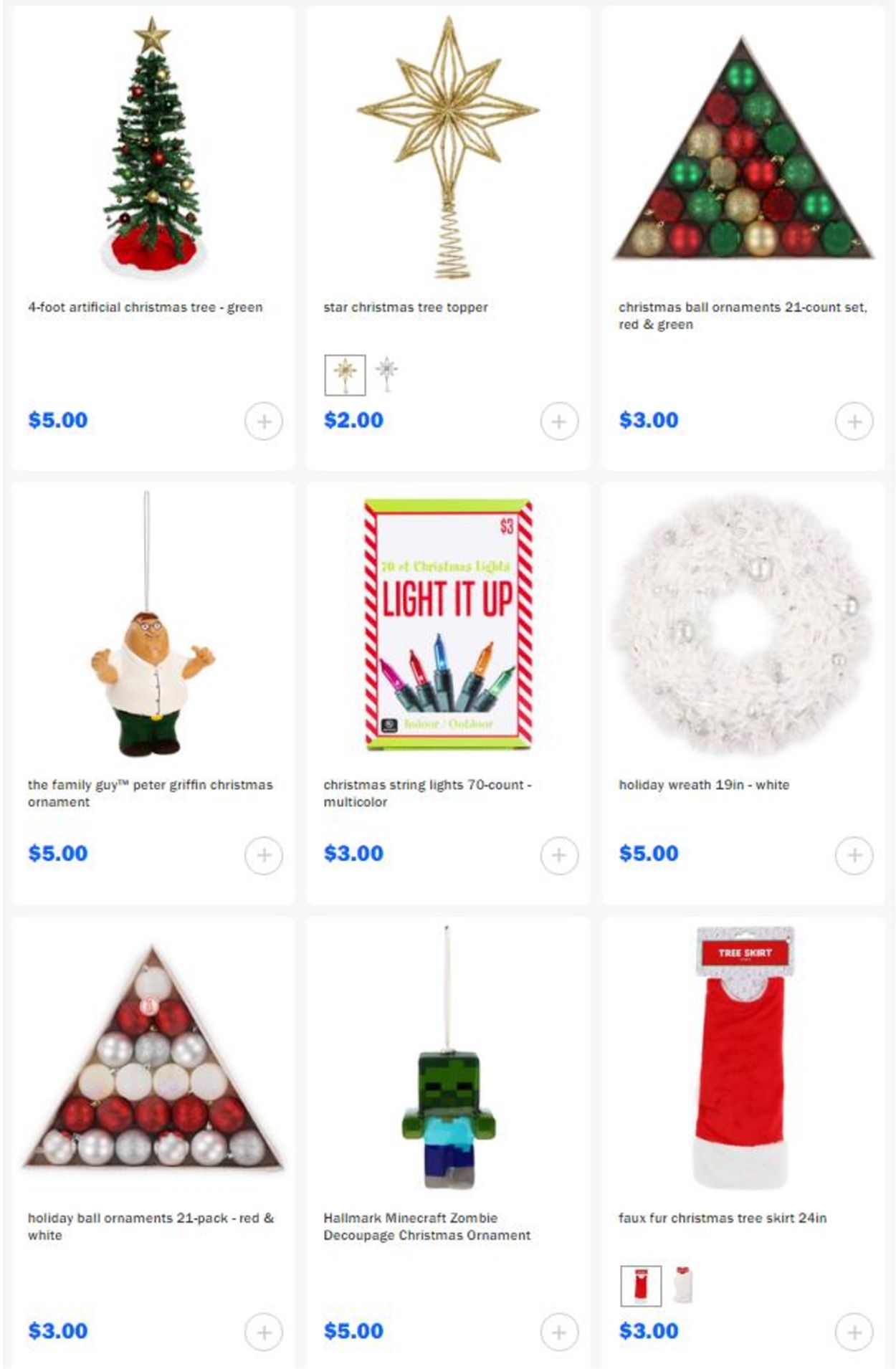This screenshot from an unidentified e-commerce website showcases an array of Christmas-themed items, organized in three neatly divided rows, with three products per row, set against a white background.

- **Top Row:**
  - **Left:** A small Christmas tree priced at $5, displayed in bold blue font.
  - **Center:** A glittering gold star tree topper ornament, available for $2.
  - **Right:** A triangular box filled with round ornaments in festive colors of green, red, and gold.

- **Middle Row:**
  - **Left:** An ornament shaped like a rotund man dressed in a white shirt and black pants.
  - **Center:** A package labeled "Light it up", containing string lights suitable for decorating a Christmas tree.
  - **Right:** A lightly colored, almost silver wreath.

- **Bottom Row:**
  - **Left:** Another triangular box of ornaments, this time in silver, red, and white.
  - **Center:** A whimsical box-shaped ornament resembling a green little man.
  - **Right:** A red Christmas tree skirt designed to be placed around the base of the tree.

Each product is distinctly visible and clearly categorized, making the shopping experience user-friendly and visually appealing.